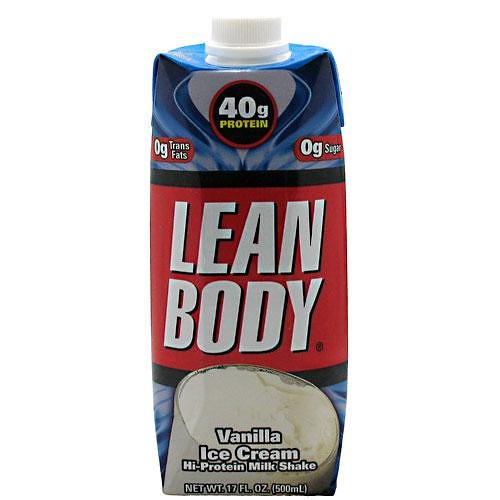The image displays a cardboard box of Lean Body Protein Shake, prominently featuring a flavor designation of "Vanilla Ice Cream High Protein Milkshake" at the bottom. Central to the box’s design is the brand name "Lean Body," which is set against a striking red square with a black border at the top and bottom. Beneath the flavor information, there is an enticing visual of a glass filled to the brim with the vanilla ice cream shake, hinting at its creamy texture and richness. The primary background color of the carton is a gradient of blue and white, giving it a clean and refreshing appearance.